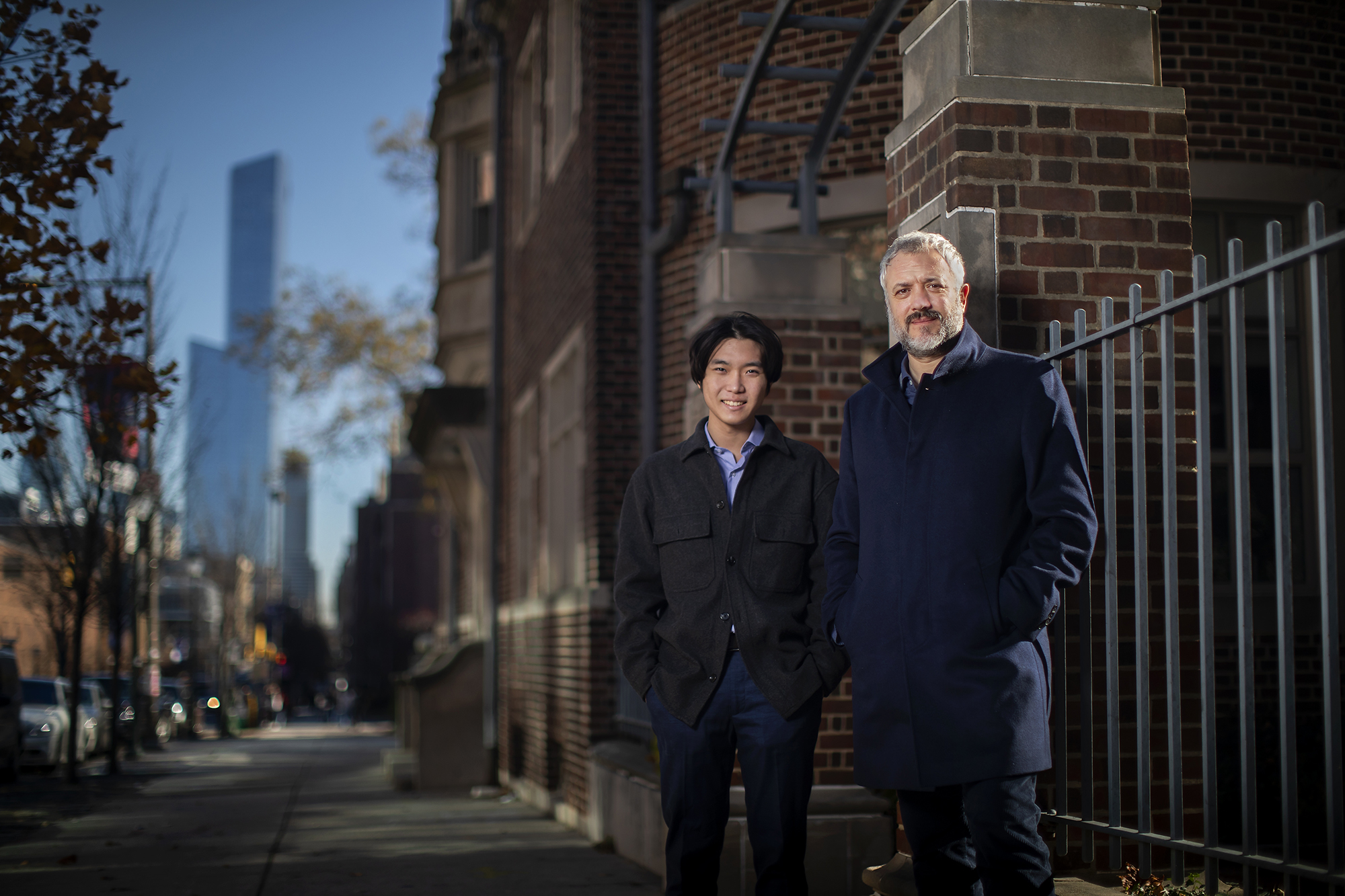In this detailed professional photograph, two men are standing on an urban sidewalk in front of a large, old-style brick building, possibly a school, church, jail, or apartment building, with black iron gates surrounding it. The older man, positioned on the right, has white hair, a white beard with a dark mustache, and is wearing a navy blue coat with matching dark blue pants. The younger man, positioned on the left, is of Asian descent, with black hair, and is dressed in a dark jacket over a blue button-down shirt and blue pants. Both men are looking directly at the camera; the younger man is smiling broadly, while the older man has a pleasant, neutral expression. The sky above is blue, and the background reveals a mix of brown and gray shorter buildings, several of which are blurred out. There is a black iron fence to the right of them, and to the left, the sidewalk is lined with trees, including one with purple leaves. A couple of bare trees and some green foliage can also be seen in the background amongst the urban skyline, which includes towering skyscrapers. The scene suggests a setting in a bustling city environment, capturing a moment of companionship between the two individuals amidst the urban backdrop.